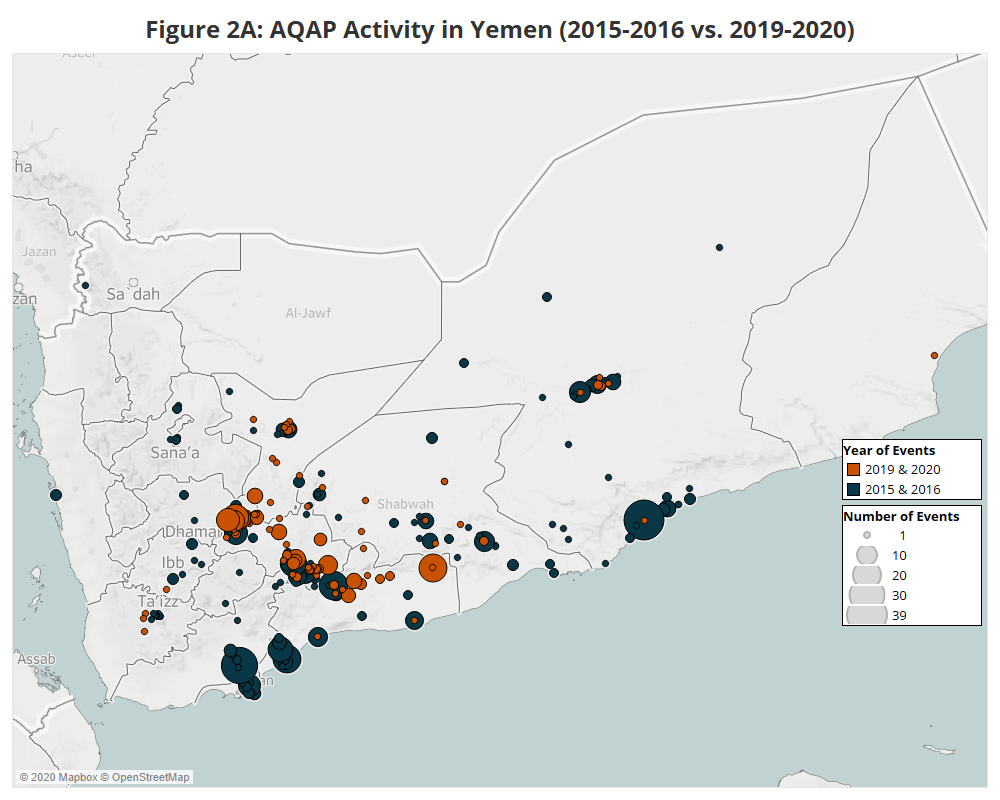The image is a detailed map of Yemen and its surrounding regions labeled "Figure 2A: AQAP Activity in Yemen 2015-2016 vs. 2019-2020." The map highlights various events over two distinct periods, utilizing a detailed legend on the right-hand side. The legend specifies that orange dots represent events from 2019-2020, while dark grey dots denote events from 2015-2016. Dots vary in size, indicating the number of events: 1, 10, 20, 30, and 39 or more. 

The map is bordered by light bluish-gray areas denoting bodies of water such as the Red Sea and parts of the Indian Ocean, with Yemen prominently displayed at the center. The events, marked by either orange or dark grey dots, predominantly cluster along the coastline, especially on the Indian Ocean side and near the southern tip of Yemen. In contrast, there is sparse activity along the Red Sea, with only one marked event. Labels for regions within Yemen are visible, resembling what might be referred to as counties or districts. Notable map details include the "Map Box and OpenStreetMaps" label in the bottom left corner, contributing to its comprehensive informational layout.